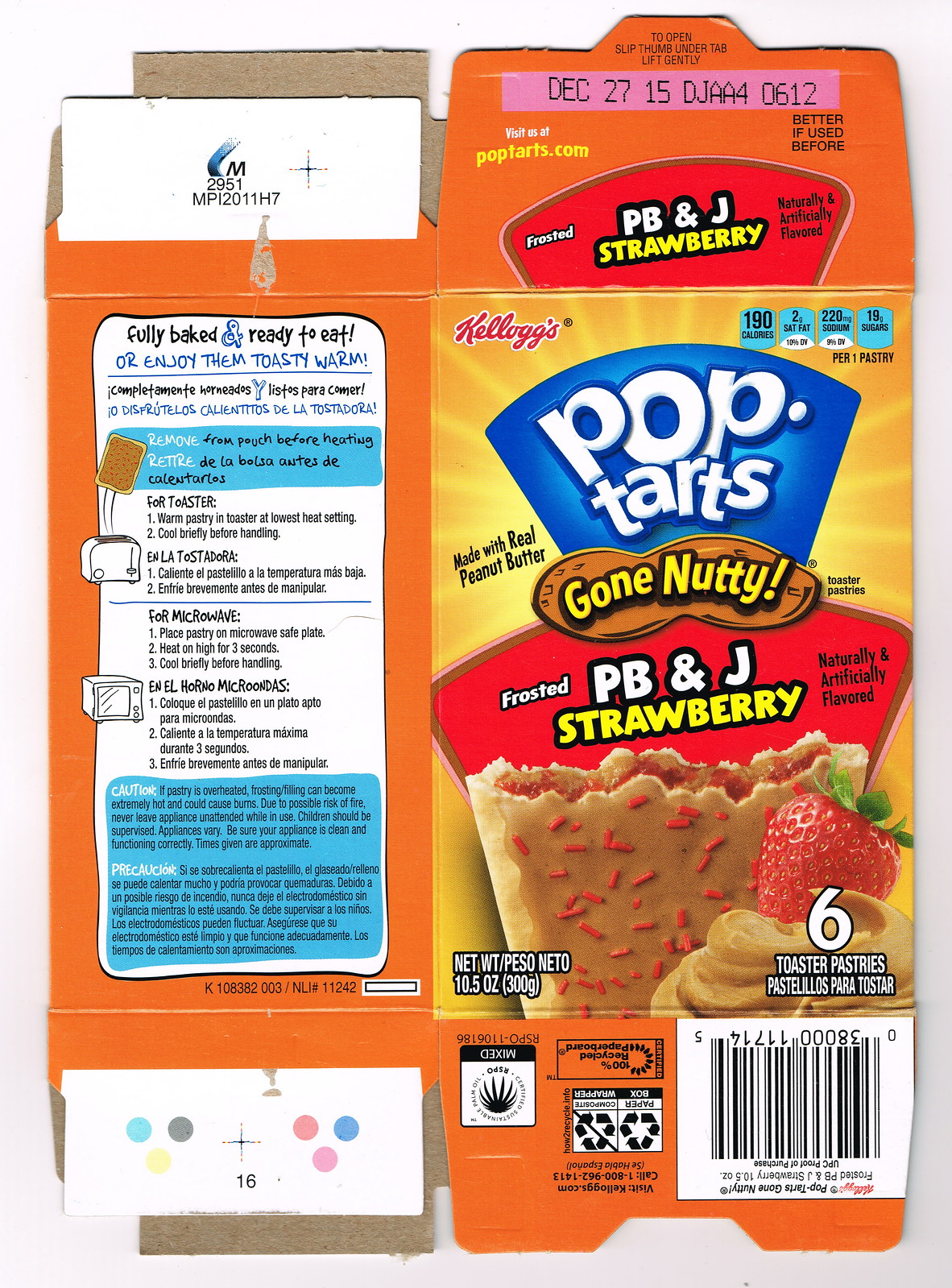This image showcases a flattened cardboard container of Pop-Tarts, allowing visibility of both the front and side of the packaging. The prominent blue logo with white lettering spells out “Pop-Tarts,” positioned just beneath the red Kellogg's logo in the upper left corner. The top of the packaging boasts the flavor, “PB&J Strawberry,” in a combination of white and yellow text set against a black or red backdrop. A pink banner atop the box highlights the expiration date, “December 27, 2015,” alongside a black printed code, “DJAA40612.”

Below the Pop-Tarts logo, the description “Gone Nutty PB&J Strawberry” appears, along with an enticing image of the Pop-Tart itself. The illustrated Pop-Tart is brown with red sprinkles, placed in front of a strawberry nestled in a mound of peanut butter. Information about the product’s quantity, “Six Toaster Pastries,” is printed in white text at the bottom of the front panel.

The left side of the box contains instructions for toasting or microwaving the Pop-Tarts, set within a predominantly white rectangle accented with blue highlights. This section also features cautionary notes, which are similarly enclosed within blue-highlighted rectangles, ensuring they stand out for consumer safety.